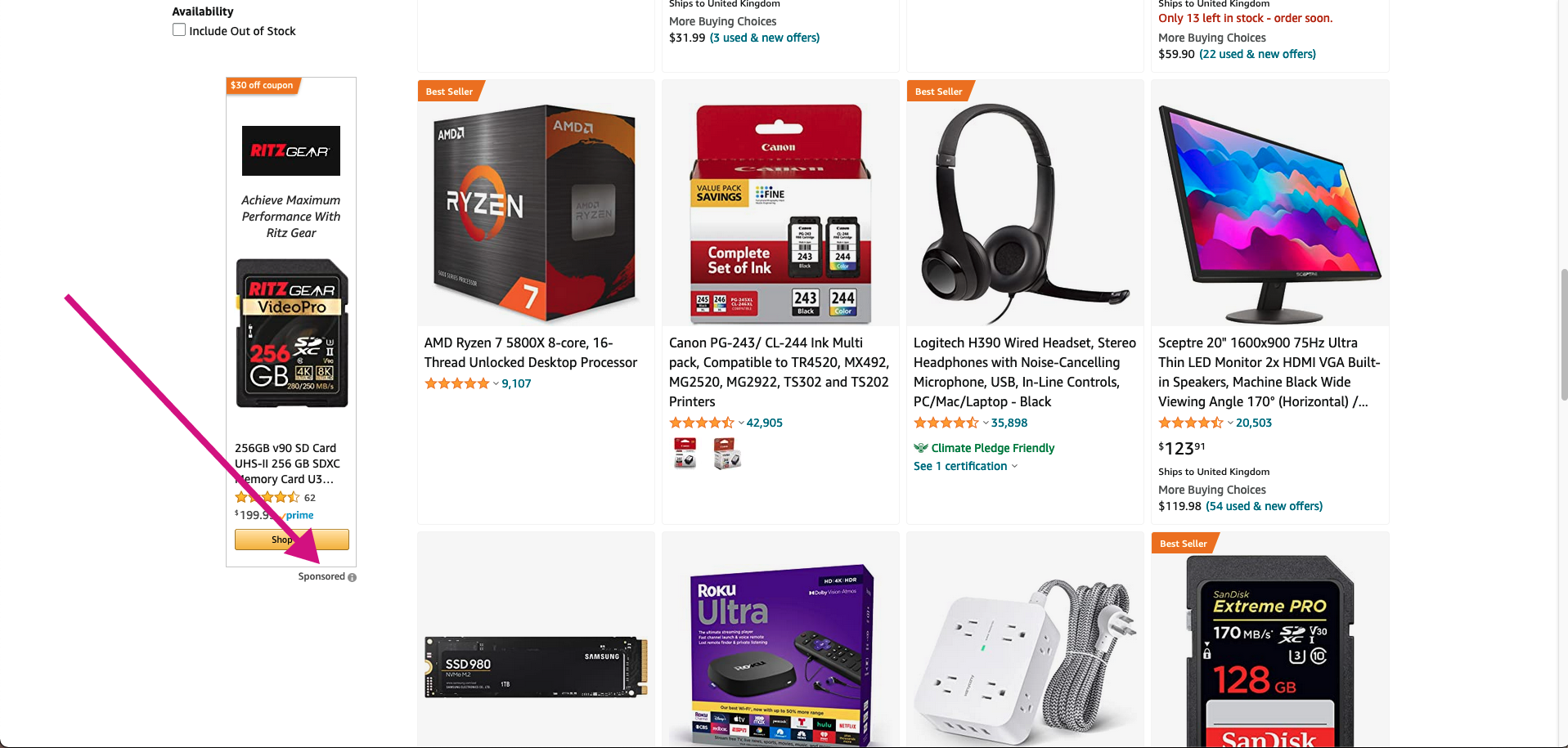The image showcases a computer screen displaying an advertisement, reminiscent of those commonly found in junk mail, promoting various computer parts. While the ad does not specify the store, it prominently features a 256GB memory card, likely meant for a phone, at the top. A green arrow highlights an illegible section of the ad, presumably guiding attention to fine print that is too small to read clearly. Additionally, the advertisement lists a Ryzen 7 CPU, various other memory cards, headphones, a sleek LED monitor, an extension cord, and other miscellaneous computer accessories. The diverse range of products suggests a focus on essential tech components and peripherals.